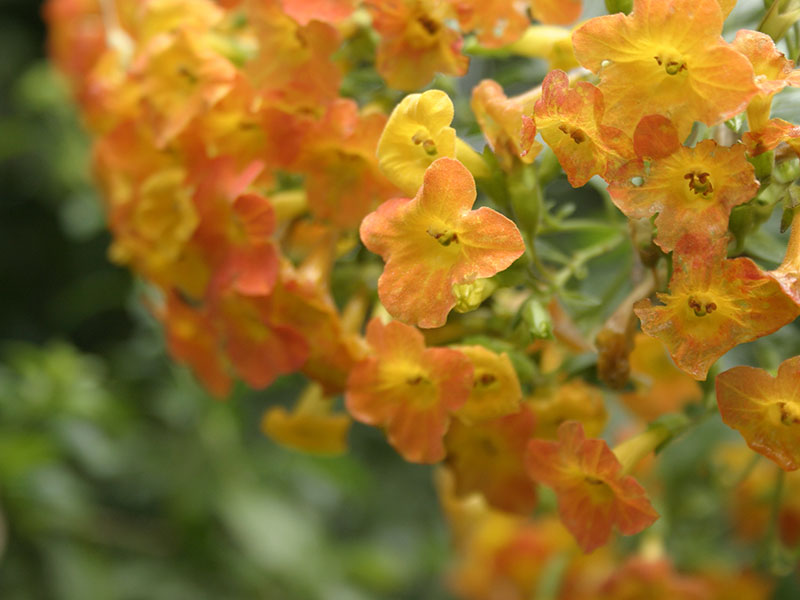This photograph beautifully captures a vibrant assembly of yellow and orange flowers, potentially resembling poppies, blooming in abundance. Dominating the right-hand side of the foreground, the flowers are depicted in sharp focus, with each blossom revealing its vivid combination of orange and yellow hues, some displaying touches of pink and red. The flowers, around the size of quarters, feature four gently curved petals and celery green stems. Visible stamen, colored red and green, hint at the flowers' delicate pollination structures. Despite the sharp foreground, the background fades into a blurred mosaic of greenery, suggesting trees or bushes basking in spring sunlight. The entire scene exudes a lively, almost painterly quality, with an estimated several dozen blooms filling the composition, transitioning to blurs toward the upper left corner. The overall rectangular image showcases the flowers in their seasonal glory, evoking a sense of both detail and the natural, unfocused beauty of a blooming landscape.